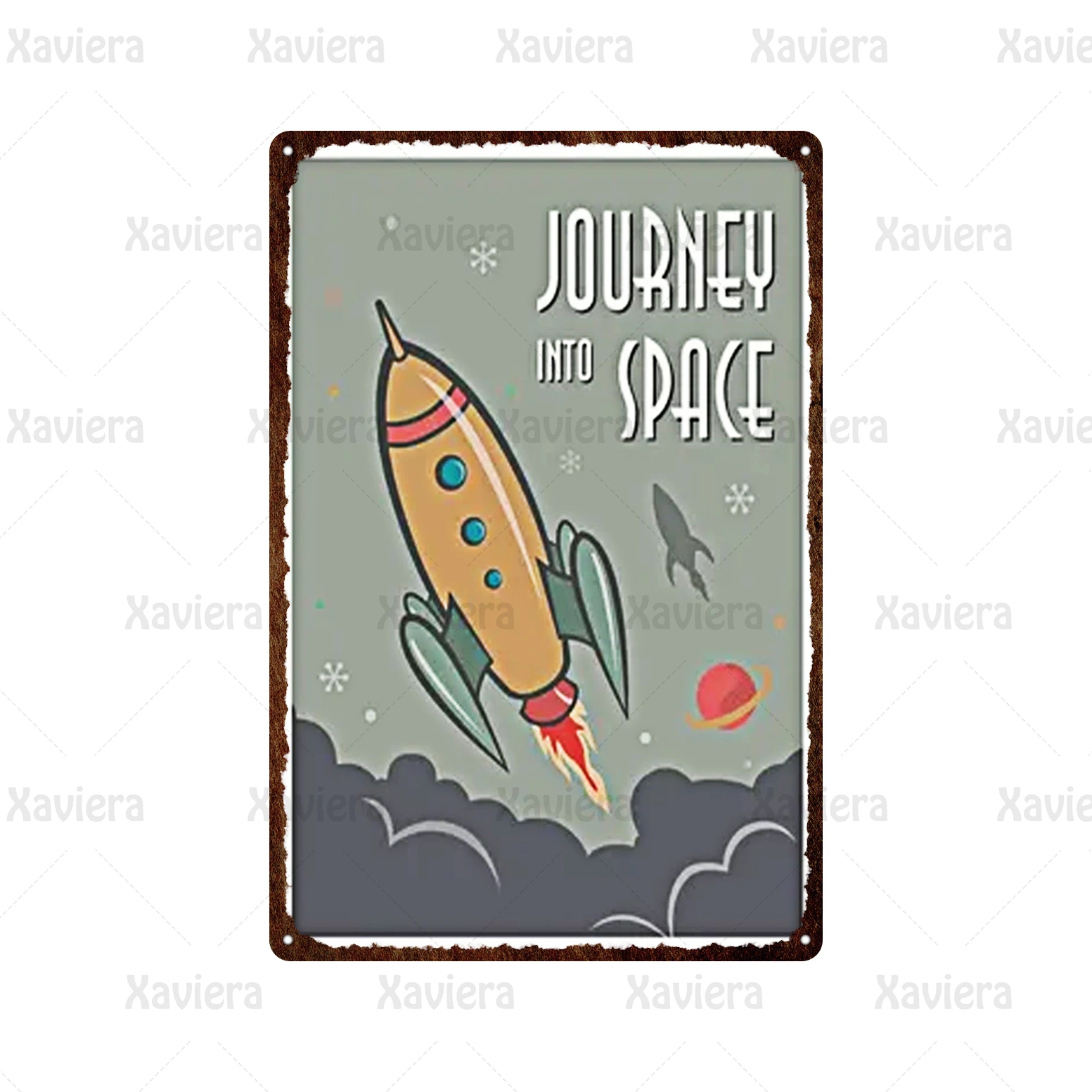The image is a commercial photograph of a rectangular metal wall print, designed for online shops, websites, or catalogs, featuring a cartoon rocket ship with a vintage 1940s-1950s science fiction aesthetic. The metal plate, placed against a solid white background which makes it appear as if it is floating in an empty void, showcases a whimsical and detailed artwork. The rocket ship, rendered in a gold color with a red stripe around its top, sports three blue windows that decrease in size from top to bottom. Its torpedo-like shape is accentuated by a sharp needle-like tip and grayish-green fin-like wings. Brilliant red and yellow flames are illustrated bursting from the rocket's base, suggesting liftoff. Below the rocket, there is a depiction of dark gray clouds and silhouetted surroundings, including a replica of the rocket and snowflake-like details. The artwork includes the text "Journey Into Space" in white, located in the top right corner. Additionally, a red planet with a yellow ring, reminiscent of Saturn, appears in the bottom right corner. A semi-transparent watermark text, spelling "X-A-V-I-E-R-A" repeatedly and interspersed with dotted gray diamond lines, overlays the entire image.